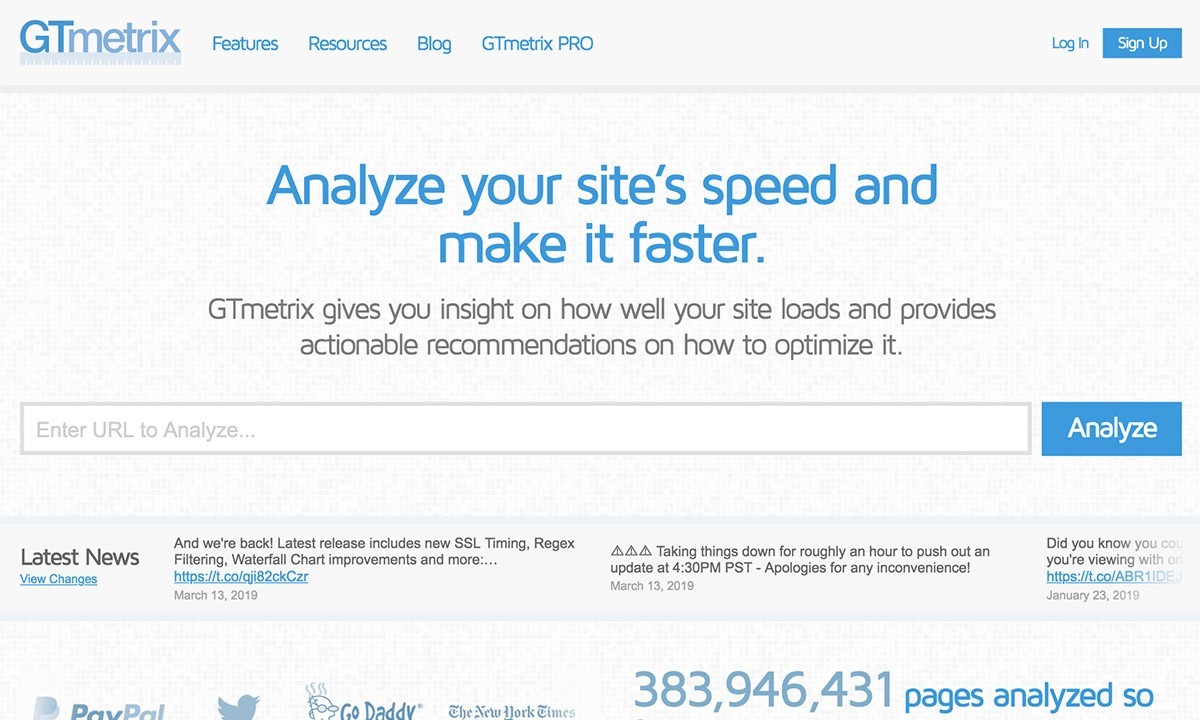This screenshot captures a web page from the GTmetrix website, characterized by a predominantly grey background with blue and black text. At the top-left corner, the GTmetrix logo is displayed with an accompanying measuring tape graphic just beneath it. The header also includes blue navigational links labeled "Features," "Resources," "Blog," and "GTmetrix Pro." On the far-right corner of the header, there are options to "Login" and a blue "Sign Up" button.

In the center of the screen, prominent blue text commands attention with the message, "Analyze your site's speed and make it faster." Below this, in black text, it explains, "GTmetrix gives you insight on how well your site loads and provides actionable recommendations on how to optimize it." Further down, there is a text box with grey placeholder text reading, "Enter URL to analyze..." accompanied by a blue "Analyze" button with white text for users to submit their site URLs.

At the bottom of the image, the section titled "Latest News" provides updates: "And we're back! Latest release includes new SSL timing, rejects filtering, waterfall chart improvements, and more," followed by a URL for more details. Adjacent to this, another update reads, "Taking things down for roughly an hour to push out an update at 4:30 pm PST. Apologies for any inconvenience."